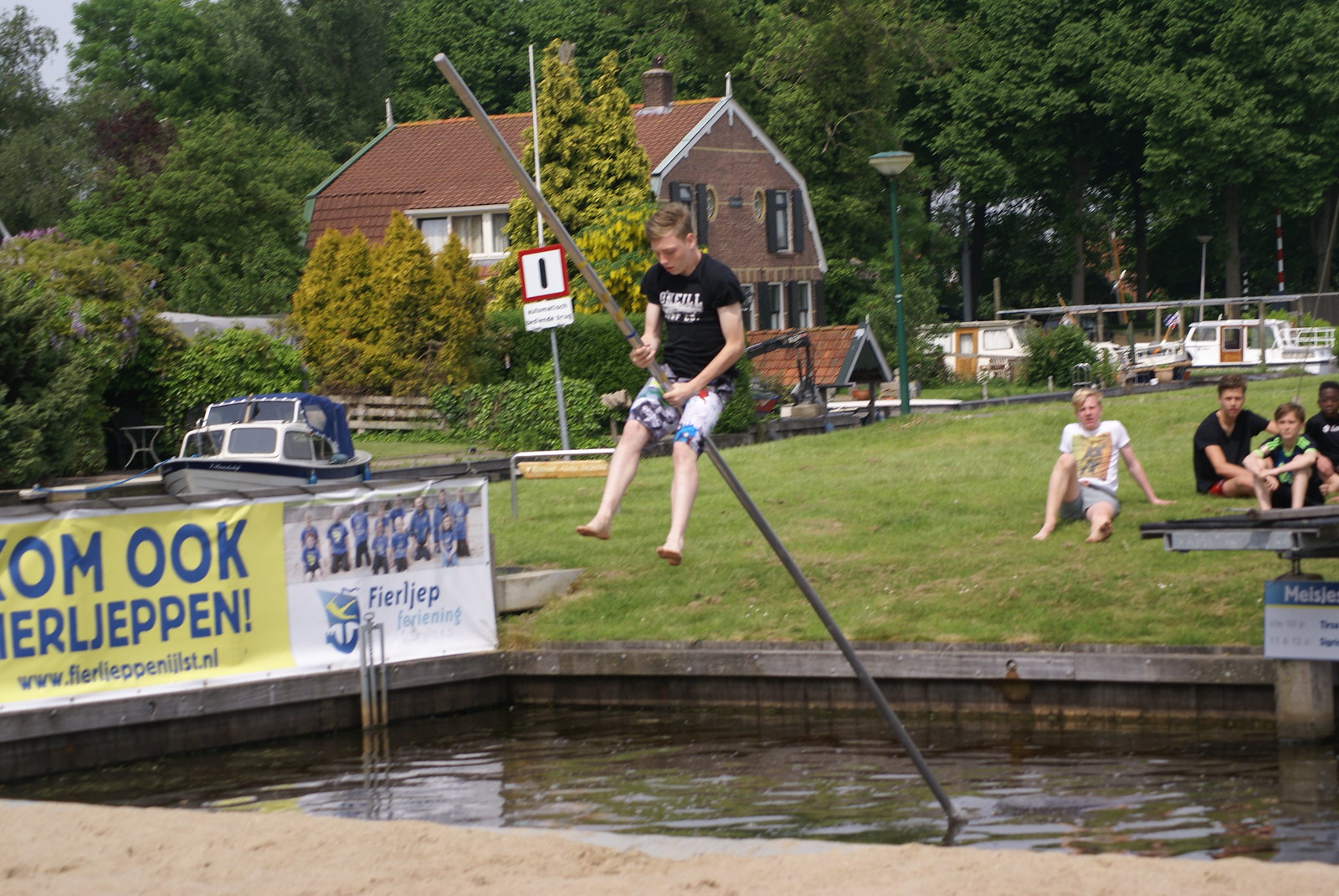In this vibrant, sunny scene, a man is captured in mid-action, balancing on a long, five-meter metal pole that extends at an angle from a square pool. He clutches the pole with both hands while positioning his knees against it, and he appears to be a white man with brownish hair, dressed in a black t-shirt adorned with white lettering and multicolored swim shorts in hues of blue, white, and black. His bare feet dangle down as he sits precariously on the pole, which is angled at approximately 45 degrees. The scene takes place on a clear, likely hot day given that everyone is dressed in t-shirts.

The pool is surrounded by a lush grass area where several people, including a group of four children, are seated, intently watching the man's daring stunt. In the background, a red brick, barn-shaped building with a brownish-red roof can be seen, adding a rustic charm to the scene. Further adding to the picturesque setting is a boat, white and blue in color, resembling a small yacht, visible in the distance.

On the left side of the image, there is a horizontal rectangular poster displaying text in what appears to be a Scandinavian language, possibly Swedish. The poster features a yellow and blue font, adding a splash of color to the scene. Additionally, a small pole with the number 'one' is present near the pool.

The entire composition is lively and engaging, with trees forming a forest-like backdrop, while a myriad of leaves hint at a rich, natural environment. The combination of human activity, architectural elements, and natural beauty makes this image rich in detail and full of life.